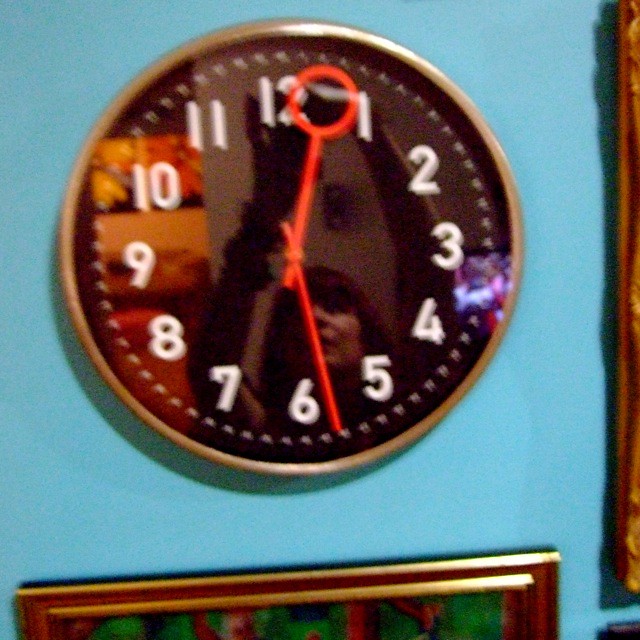The image showcases a slightly blurred picture of a round wall clock with a distinct copper or gold-colored rim. The clock is mounted on a light blue wall. The clock face is black, adorned with white numbers and markings, and protected by a glass cover that reflects a woman reaching up, along with some background items. The hour hand is red with a large circle at the end, while the minute hand is a simple red straight line. Below and to the right of the clock, there is a rectangular picture frame in a gold or light wooden color, adding a touch of elegance to the scene.